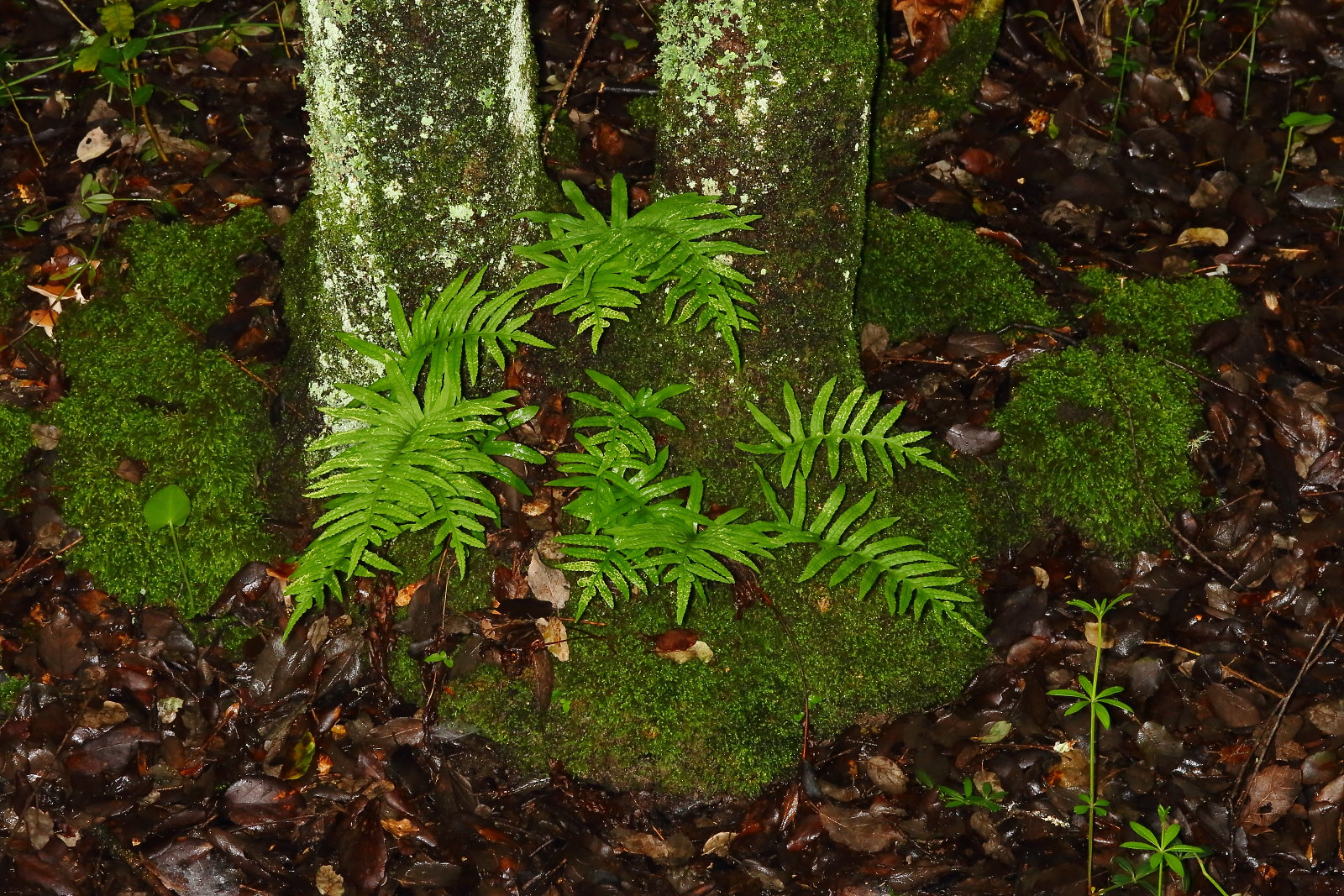This photograph captures a rich, wooded area featuring a close-up of the bases of two trees enveloped in a thick layer of green moss. The ground around the trees is densely covered with dark brown, almost blackish dead leaves, obscuring much of the dirt and stone beneath. Both trees display patches of white fungus or mold contrasting against their primarily greenish-brown trunks. The moss on the trees transitions to lighter, shinier patches, possibly indicating fresher growth. From this moss, vibrant light green ferns sprout, adding to the lushness of the scene. The entire area appears damp, likely from recent rain, enhancing the vibrancy of the foliage. While the moss-covered areas display a sickly greenish-gray tinge, the overall impression is one of thriving, wet woodland ecology.